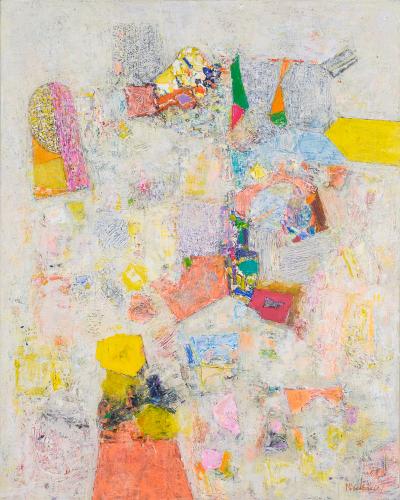The image depicted appears to be a low-resolution photograph of an abstract, surrealistic painting rendered in what seems to be oil on paper. The overall palette is composed of light, almost washed-out colors, including shades of light blue-gray, light red, yellow, green, gray, teal, purple, bright pink, and orange, set against a beige or grayish backdrop. The painting features an array of amorphic and geometric shapes that are not perfectly organized, giving it a chaotic and playful feel. Notable is a larger, solid figure at the bottom, characterized by a white head and hands, enveloped in a gray cloak-like shape. Some shapes in the painting vaguely resemble a question mark, adding to its abstract nature. Despite the playful use of colors, the overall impression is somewhat fuzzy and dull due to the toned-down hues. A signature is present in the bottom right corner, though it is not legible in the current image quality.